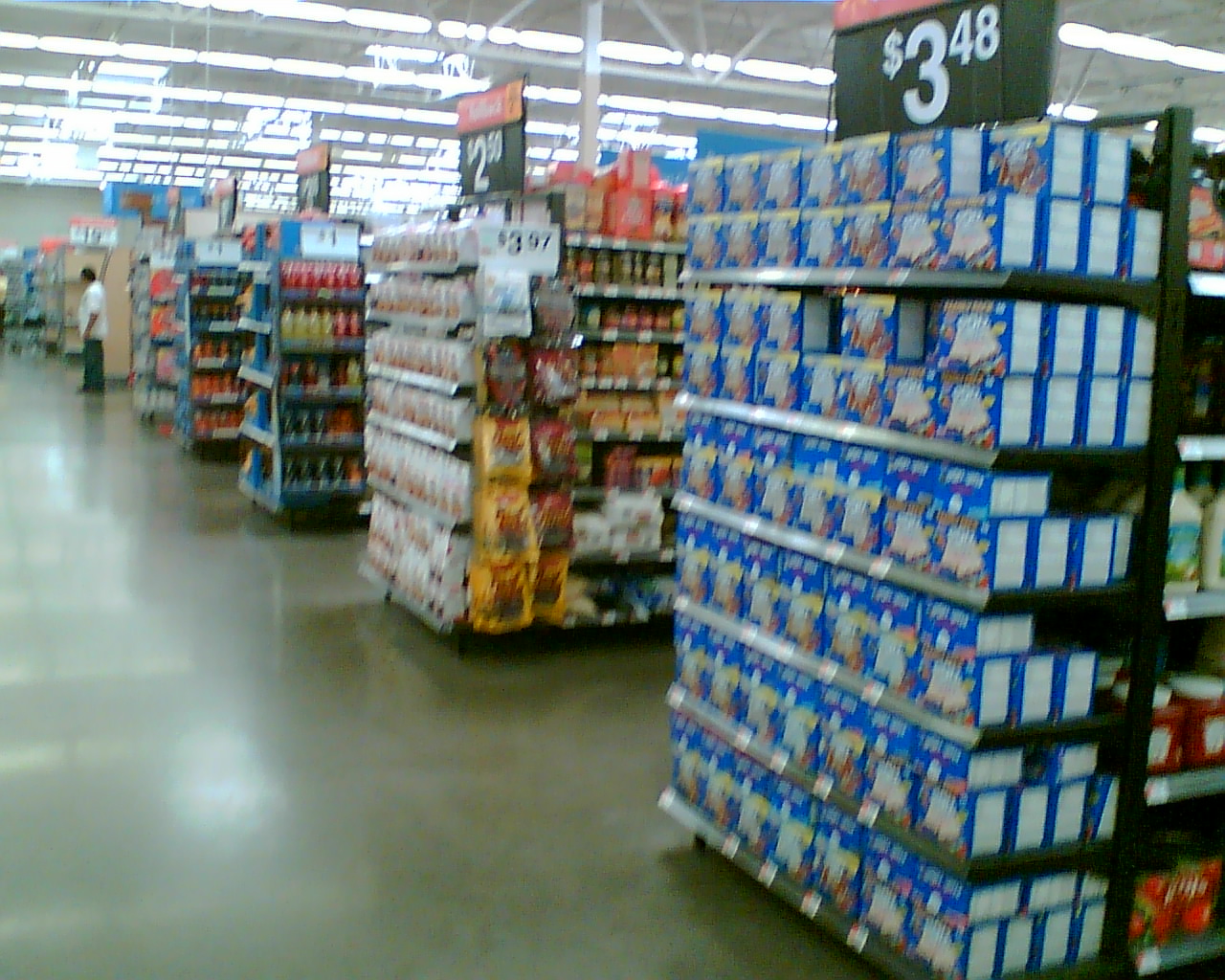In this image, taken from the center aisle of a grocery store, we observe several end caps of various aisles, each stocked with diverse items. The store's cement floor is light gray, illuminated by bright white fluorescent lighting suspended from the ceiling. On the first aisle to the right, there are fully stocked shelves of cereal boxes. These boxes are prominently blue with white sides and feature a cartoon character in the center, priced at $3.48. Further down the same aisle, interspersed boxes have been taken, leaving some gaps on the shelf. Next to this aisle, there's another featuring spices in visually striking orange, blue, yellow, and red packaging, with the price marked at $3.97. Additionally, white boxes priced at $2.50 are visible on an adjacent aisle. Alongside, there is an aisle displaying various drinks and juices with a price tag of $1. Amidst the aisles, a person wearing a white shirt and dark pants stands in the distance, adding a human element to the bustling store environment. While some of the image is slightly out of focus, the price tags and general layout of the grocery items are discernible.